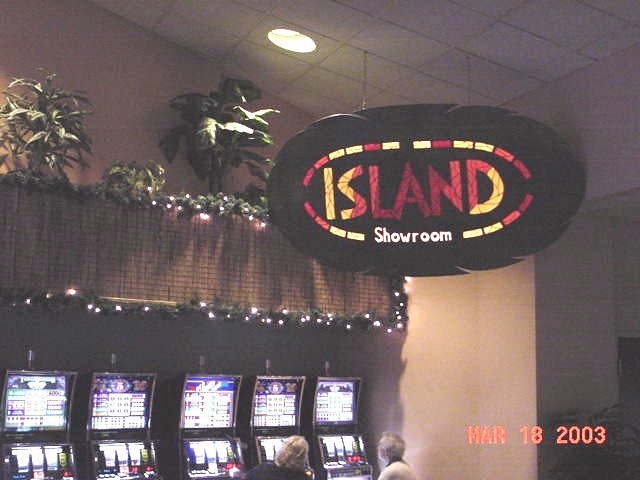In this vibrant photograph capturing the essence of a bustling casino, we see a row of five slot machines aligned against a tan-colored wall, each adorned with intricate designs. Two individuals, both with grayish-colored hair, are engrossed in their respective games. One is clad in a crisp white shirt, and the other sports a sleek black shirt. The upper left corner of the image features decorations inspired by an island theme, with palm tree motifs adding a touch of tropical flair. The sign fronts have a charming wicker-style design, enhancing the relaxed ambiance. Above, a white drop ceiling supports a prominent black oval sign, emblazoned with the words "Island Showroom" in a vibrant palette of yellow and red. The sign is also accented with a dotted line of the same colors, drawing attention to this entertainment hotspot. The lower right corner of the photograph displays the date, March 18th, 2003, marking the moment this lively scene was captured.